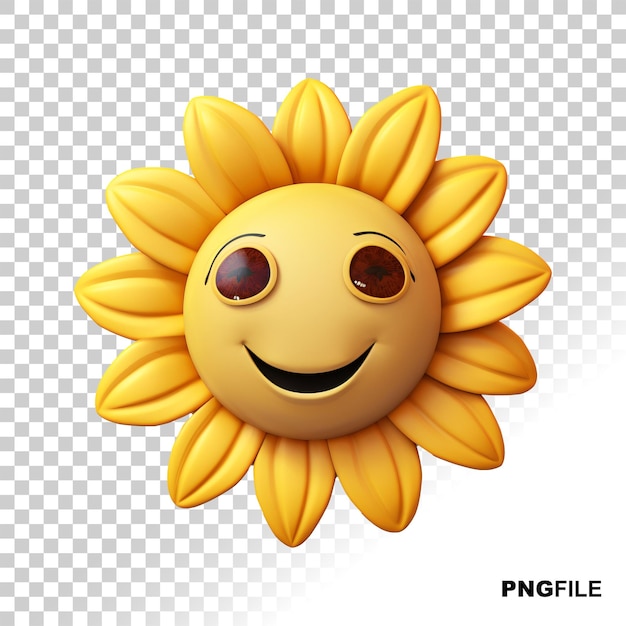The image is a computer-generated vector graphic of a vibrant sunflower with an emoji-like face at its center. The background features a gray-and-white checkerboard pattern that indicates a transparent PNG file, with "PNG FILE" subtly marked in the bottom right corner. The sunflower's central yellow sphere, or face, showcases expressive brown eyes encircled by yellow, thick black eyebrows, and a wide, open black smile, though it lacks a nose. The sunflower's petals are skillfully shaded, radiating outward in layers, and exhibit well-defined lines. The checkerboard background subtly fades from top to bottom, becoming completely white by the lower right corner. This playful and detailed artwork combines vivid colors and meticulous shading, illustrating a lively and cheerful sunflower emoji against a seemingly transparent backdrop.